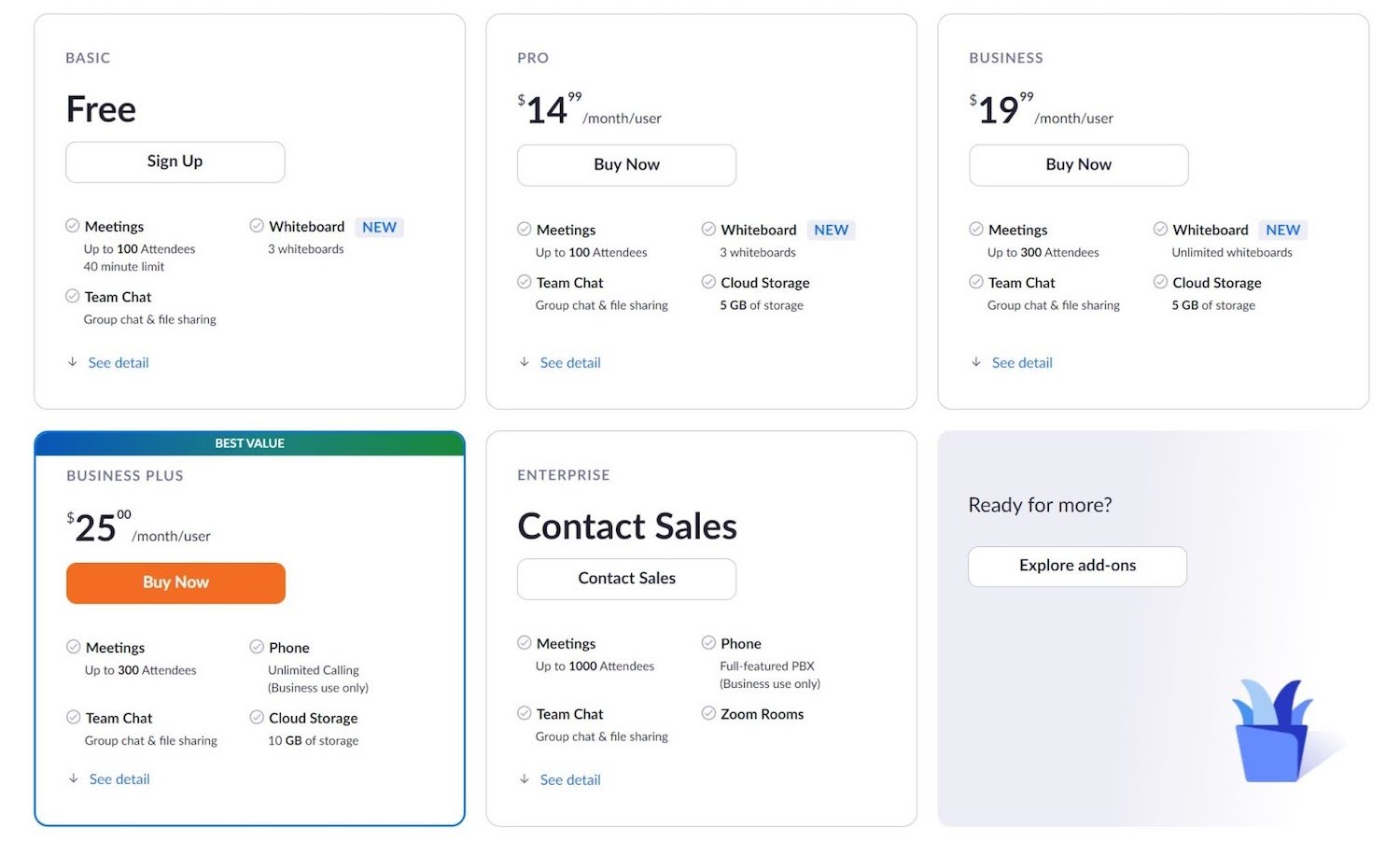The image showcases various business plans available for Zoom, detailing the pricing and features associated with each tier. There are six boxes in total, displayed against a backdrop of a gray background with a blue abstract image of a plant in the bottom right corner. Five of these boxes feature a white background and are filled with information about different subscription plans. 

1. **Basic Plan (Free)**
   - Meetings for up to 100 attendees
   - 40-minute time limit
   - Team chat, group chat, and file sharing
   - Whiteboard access with three whiteboards (new feature)
   - Option to "See Details"

2. **Pro Membership ($14.99 per month/user)**
   - Meetings for up to 100 attendees
   - Team chat, group chat, and file sharing
   - Whiteboard access with three whiteboards (new feature)
   - Cloud storage of 5 GB
   - Option to "See Details" and "Buy Now"

3. **Business Plan ($19.99 per month/user)**
   - Meetings for up to 300 attendees
   - Team chat, group chat, and file sharing
   - Unlimited whiteboard access
   - Cloud storage of 5 GB
   - Option to "See Details" and "Buy Now"

4. **Best Value Business Plan ($25 per month/user)**
   - Meetings for up to 300 attendees
   - Team chat, group chat, and file sharing
   - Unlimited whiteboard access
   - Phone service with unlimited calling for business use only
   - Cloud storage of 10 GB
   - Option to "See Details" and "Buy Now"

5. **Enterprise Plan**
   - Contact sales for pricing details
   - Meetings for up to 1,000 attendees
   - Team chat, group chat, and file sharing
   - Phone service with full-featured PBX for business use only
   - Zoom Rooms access
   - Option to "See Details" and "Contact Sales"

6. The bottom right box simply states, "Ready for more? Explore add-ons," pointing users towards additional functionalities they can purchase.

This structured overview helps users understand the breakdown of features corresponding to each pricing tier and identify the plan that best suits their needs.